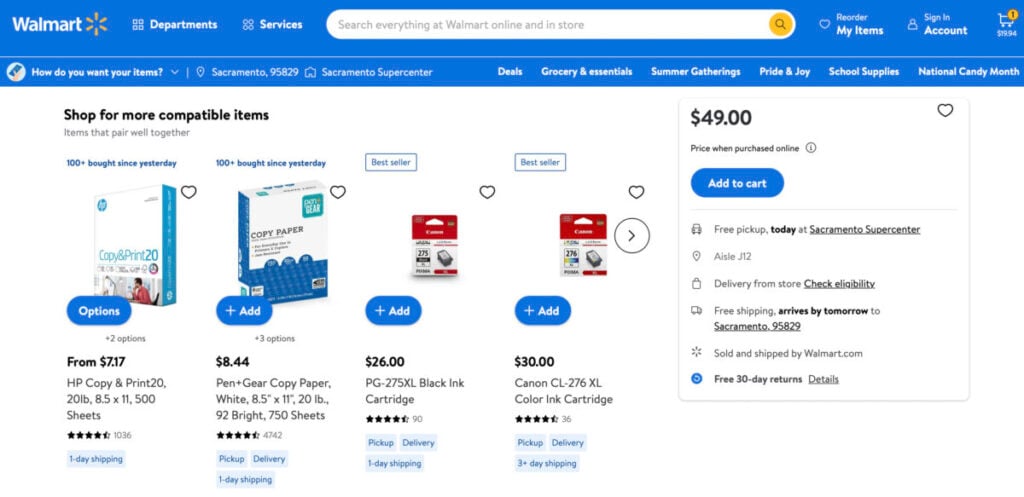This screenshot captures a Walmart web page, prominently featuring the retailer's recognizable branding. In the upper left corner, "Walmart" is displayed alongside the iconic yellow sunburst logo. Adjacent to this, a horizontal blue navigation bar spans the top of the page, containing tabs for "Departments" and "Services." Centrally located within this bar is a white search box for user queries.

To the right of the search bar, options for "My Items," "Sign In Account," and a shopping cart icon are visible. The shopping cart icon has a yellow circle with the number "1," indicating one item currently in the cart.

Below the navigation bar, the focal point shifts to products related to office supplies. On the left side, two types of computer paper in blue and white packaging are displayed, both labeled for copying and printing purposes. Centrally positioned is a red and white Canon black ink cartridge.

On the far right, detailed purchasing information for the Canon ink cartridge is provided. The price is listed as $49 with a note specifying "Price when purchased online." Below the price is a blue "Add to Cart" button. Additional details outline various delivery and pickup options, including free pickup at the Sacramento Supercenter (ILJ12), delivery from the store availability, free shipping estimated to arrive by tomorrow, and terms of the free 30-day return policy, all sold and shipped by Walmart.com.

Overall, this image illustrates a typical online shopping experience on Walmart's website, highlighting available products and detailed purchase options.